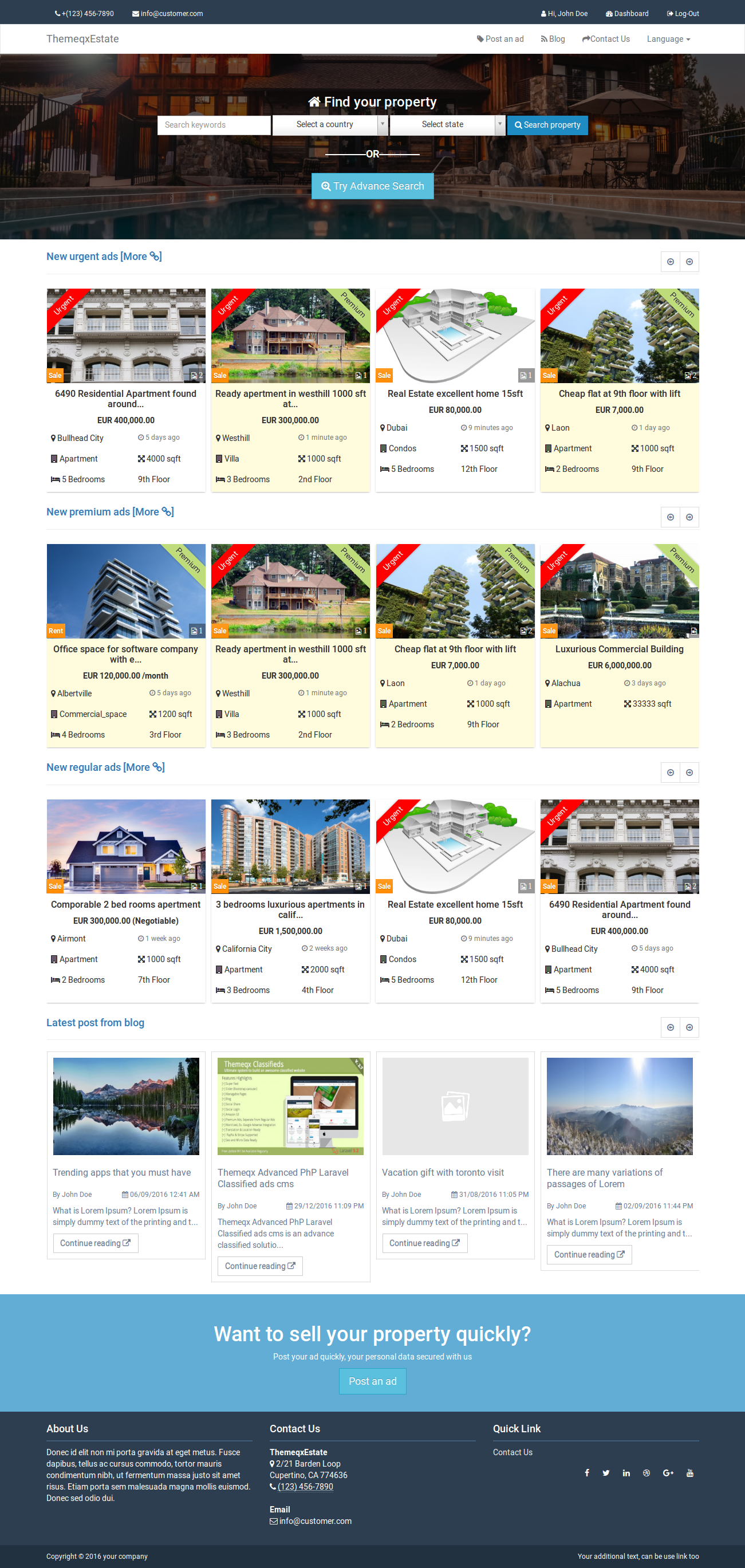The image depicts a somewhat small and blurry image of a property search webpage. The top section of the image features a black border with the phrase "Find Your Property" prominently displayed. Below this header, the layout includes a text input box on the left and a drop-down menu on the right, followed by another drop-down menu beneath the first one. Two blue buttons are stacked below these forms.

The main section of the image has a white background and displays several property thumbnails. These thumbnails include images of homes, which appear to be apartment condos in many cases, and some are merely architectural blueprints. One thumbnail lacks any image altogether. Each thumbnail includes a description underneath and some display a small red ribbon on the top left, likely indicating the property is on sale. At the bottom of the image, a light blue box invites users to "Sell Your Property Quickly," with a dark blue box positioned below this call-to-action.